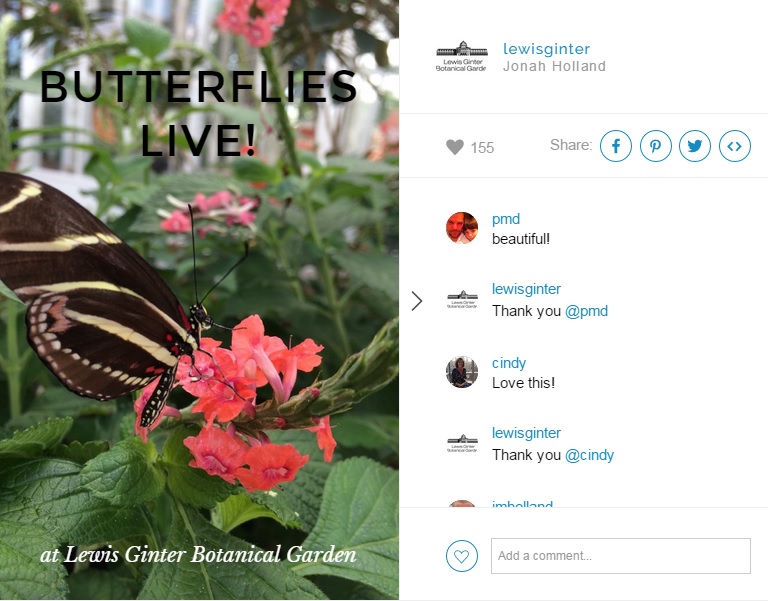A screenshot displaying the vibrant ecosystem at Lewis Ginter Botanical Gardens reveals a beautiful brown and white striped butterfly perched delicately on green-leafed plants adorned with pink flowers. The image, showcased by Jonah Holland, has garnered 165 hearts and is widely shared across social platforms such as Facebook, Pinterest, and Twitter. The screenshot also includes comments from users: PMD, who has a profile picture featuring a man with a child, praises the scene with "beautiful Lewis Ginter, thank you." Another user, Cindy, shown wearing a black shirt, expresses her love for the place. A blue circle with a heart icon and a gray square labeled "add comment" are visible, set against a clean white background.